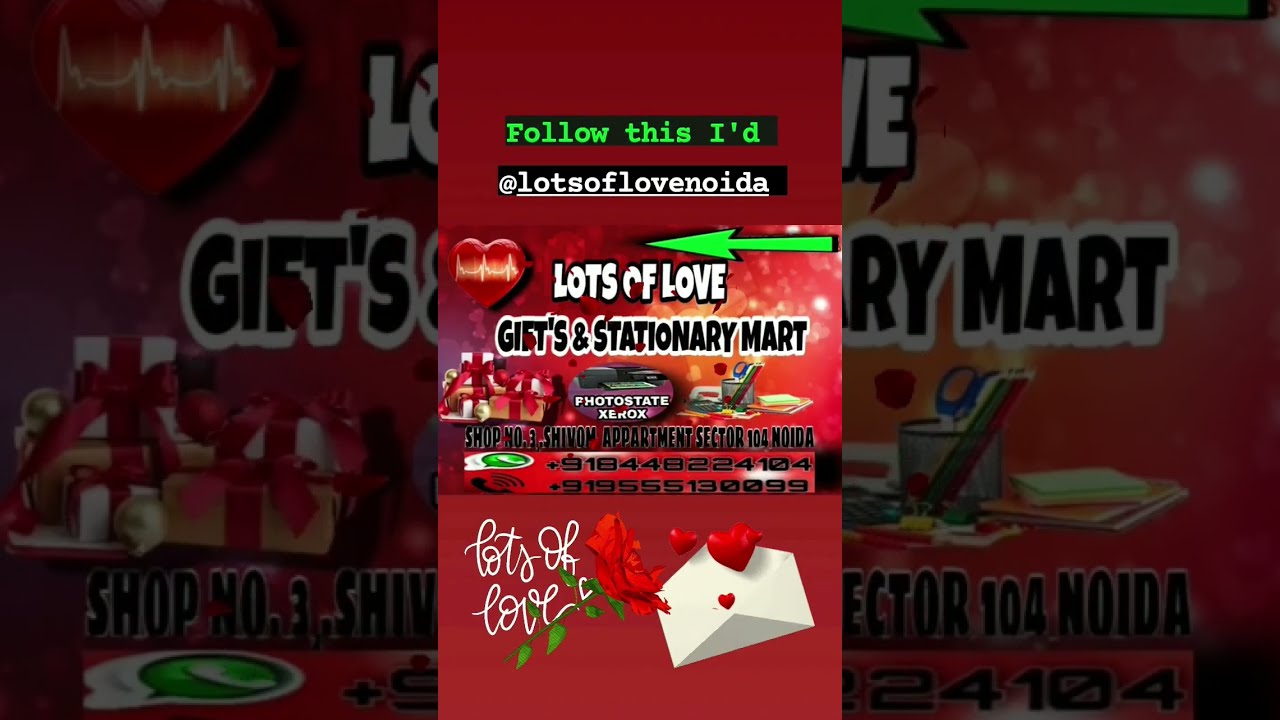The image is an advertisement with a primary focus on the middle third, presented on a red background. The top section features a black box with neon green letters stating "Follow this I'd" and another black box below it with white lettering displaying the social media handle "@LotsOfLoveNoida". A green arrow points to the left towards a red heart graphic that has a white heartbeat line, reminiscent of an EKG pattern. 

Beneath these elements, the advertisement prominently showcases the text "Lots of Love, Gifts, and Stationery Mart" with "Lots of Love" in white letters and "Gifts and Stationery Mart" in black font with a white border. Centrally positioned within an oval shape, there is an image of a Xerox machine with the label "Photo State Xerox" included.

Towards the bottom, a whimsical design includes "Lots of Love" written in cursive script, a white envelope with red hearts emerging from it, and a rose positioned to the left of the envelope. The entire advertisement is framed by a duplicated, shadowed, larger version of the image that adds depth and dimension to the presentation.